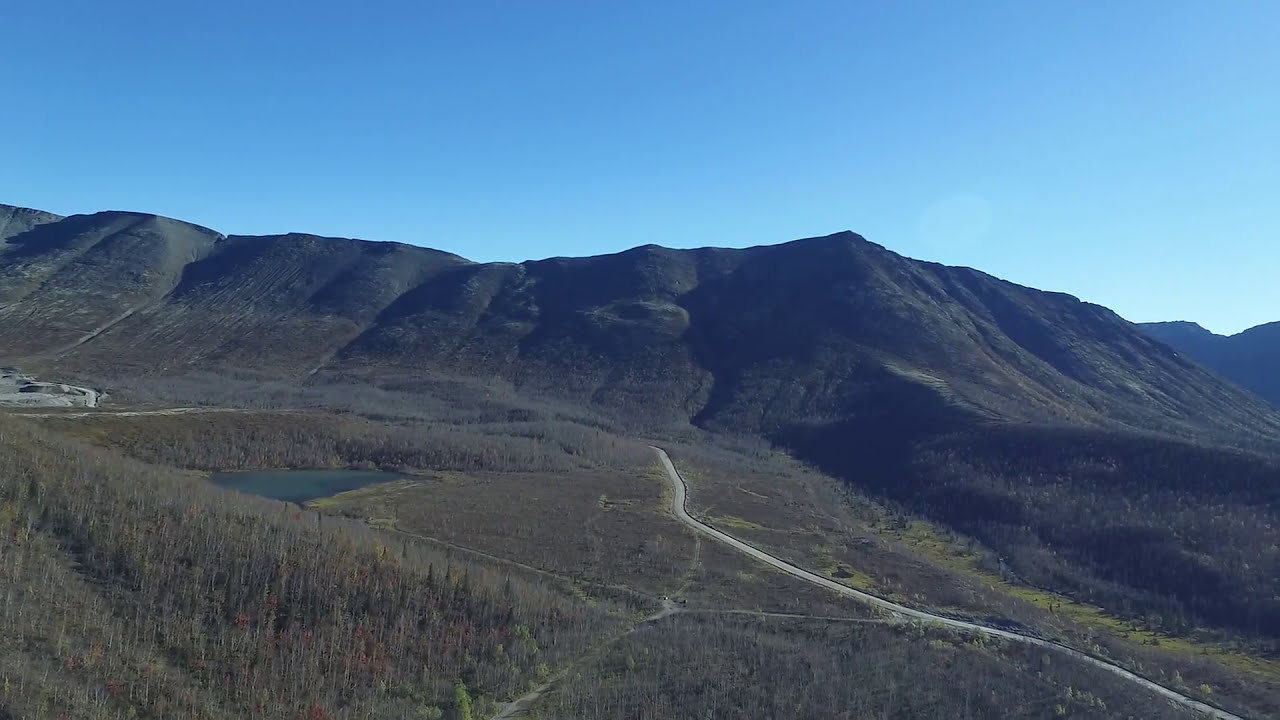In this image, an aerial perspective reveals a tranquil natural scene bathed in daylight. Dominating the center, brown mountains rise with gentle slopes and flatter peaks, framed by a clear, light blue sky that occupies the top third of the composition. The mountains gracefully transition into hilly terrain adorned with bare trees, hinting at late fall, their subdued browns and grays interspersed with the remnants of grass.

In the lower half, a serene dark blue lake rests towards the left side, bordered by a cement road that winds around it and extends from a cemented area at the bottom left corner. This road subtly transitions from the lower right corner in a 45-degree angle, gradually disappearing into the center of the image near the mountain base. The surrounding landscape is dotted with leafless trees, creating a tapestry of earth tones harmonized by the cool blue hues of the lake and sky.